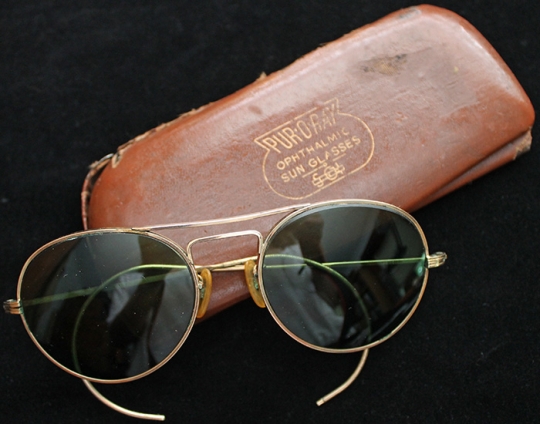A pair of vintage sunglasses with thin, gold wire frames and dark, circular lenses are carefully placed on a worn, brown leather case. The case is noticeably aged, with frayed edges, dings, dents, and a prominent black scuff mark on the top right. Embossed in gold lettering on the case are the words "Pure O-Ray Ophthalmic Sunglasses," along with a small design detail at the bottom. The scene is set against a stark black background, providing a striking contrast that highlights the sunglasses and their case. In the reflective lenses, a faint glimpse of the person taking the picture can be seen, wearing a white shirt.